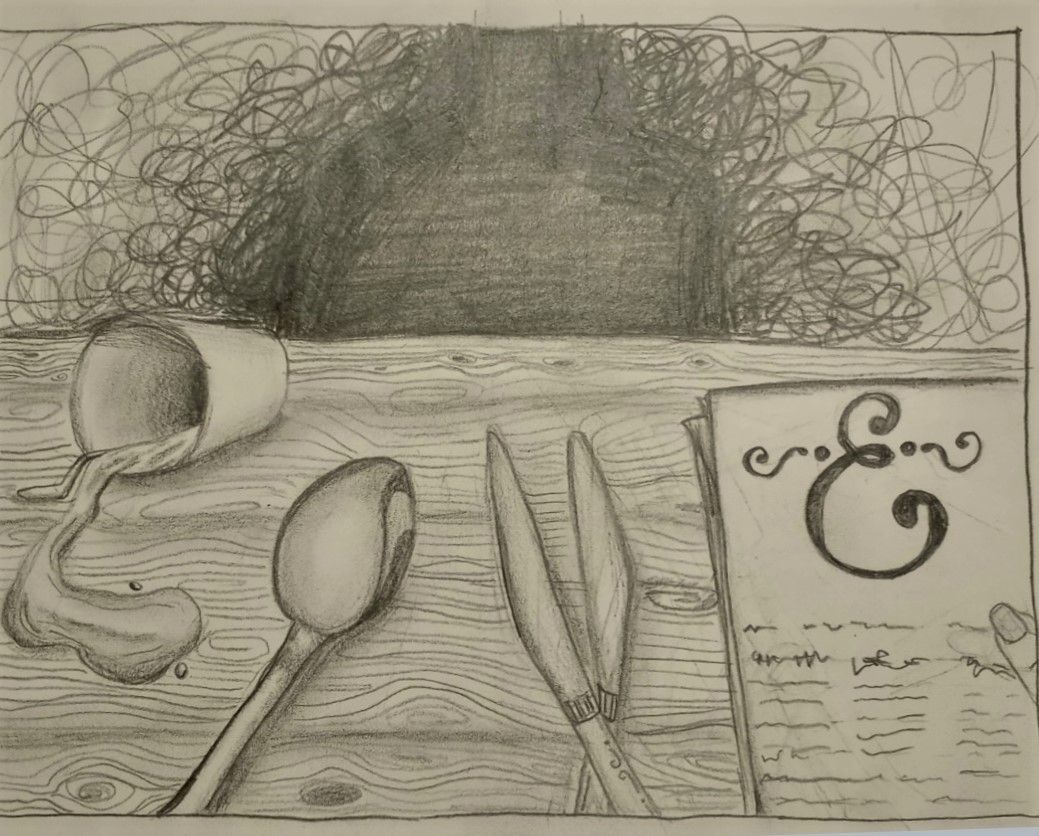The image is a detailed black and white pencil drawing set on an off-white or slate gray background. The drawing features the bottom half of a scene with a wooden restaurant table. On the table, there's an overturned cup with spilled liquid, likely milk, illustrated with subtle pencil shadings. Next to the cup, there's a large spoon, two knives crossing each other, and a pair of tongs or scissors. A menu lies to the right, with “E” written in fancy calligraphy and three columns of squiggly lines representing menu items, and a finger holding it. Above the table, squiggly lines and shaded areas create the impression of a person with long curly hair, possibly a bust, seen in the background. The overall artwork showcases skilled pencil techniques, highlighting texture and shading.